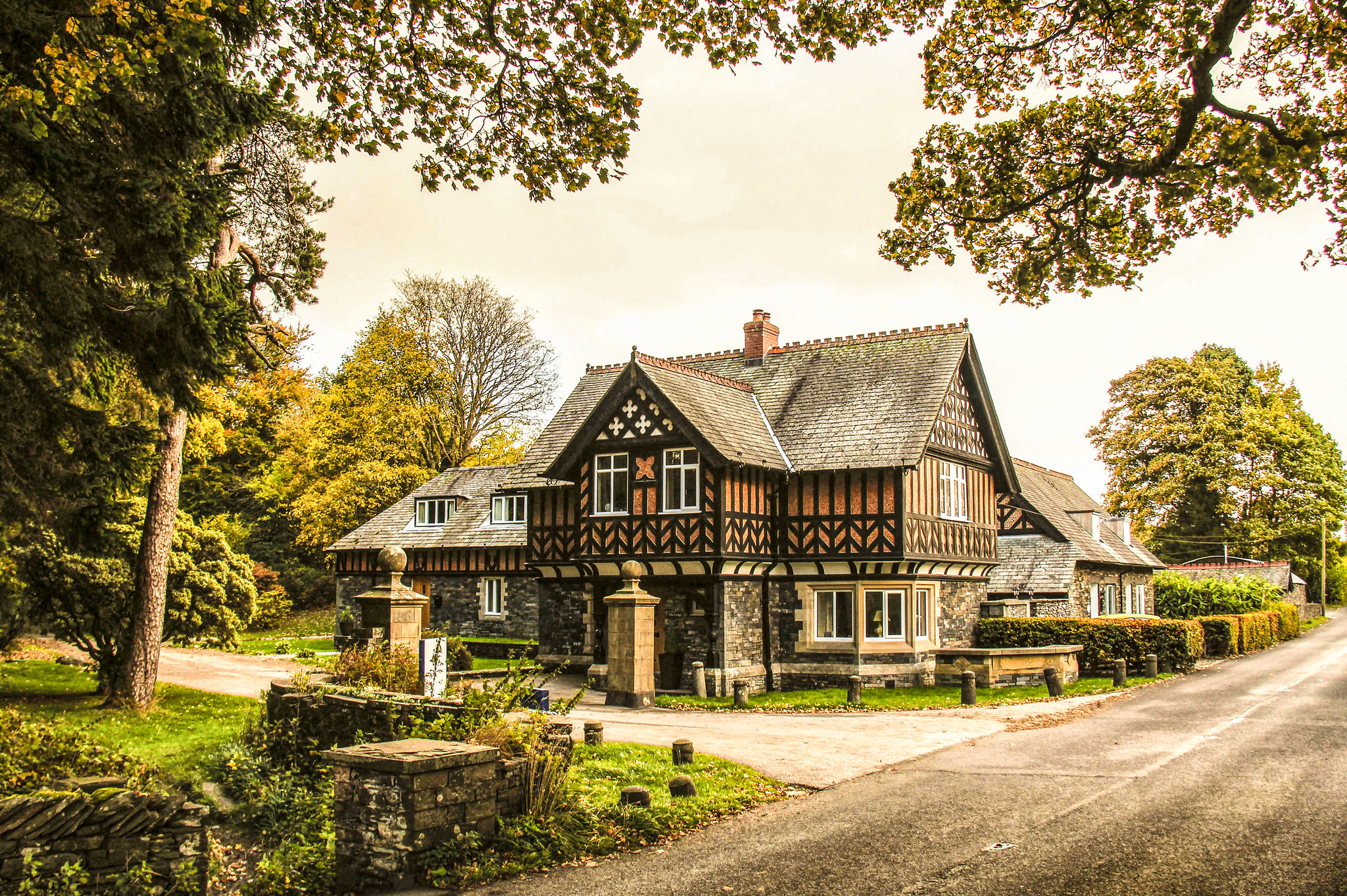A picturesque, antique English home stands majestically at the junction of a quiet side street and a main road. The charming two-story house boasts an elegant contrast of materials: the upper floor showcases rich, brownish wooden walls, while the sturdy lower floor is constructed from meticulously crafted stone. The scene is enveloped in the soft light of the late afternoon, casting gentle shadows and adding a serene ambiance. Majestic trees flank both sides of the image, their lush foliage providing a natural frame for the house. A quaint stone wall runs parallel to the main road, while dense shrubbery encircles the backyard, ensuring a sense of seclusion and privacy for the residents. The timeless beauty and intricate details of the residence are the focal points of this tranquil landscape.